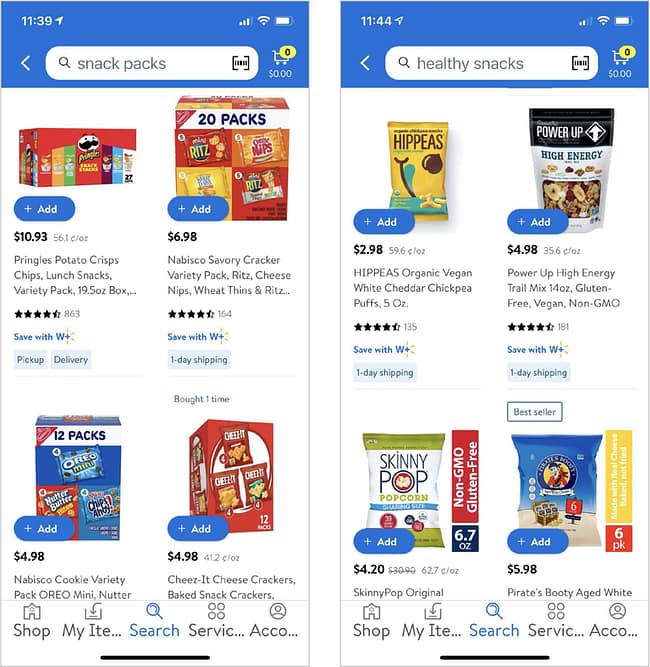**Detailed Description:**

The image consists of two screenshots taken on a mobile phone. On both screenshots, the top bar displays typical phone status icons, including the service indicator, Wi-Fi indicator, and battery level. The screenshot on the left shows the time as 11:39, while the one on the right displays the time as 11:44.

Below the top bar, each screenshot features a search bar with different queries. The left screenshot has “snack packs” typed into the search bar, while the right one displays “healthy snacks”. Both images also show an empty shopping cart, indicating that no products have been added to it.

The search results are shown beneath the search bars in both screenshots. On the left, the results include:
- Pringles Potato Crisps for $10.93
- Nabisco Savory Crackers for $6.98
- Nabisco Cookie Variety for $4.98
- Cheez-It Cheese Crackers for $4.98

In the right screenshot, the search results listed are:
- Hippies Organic Vegan for $2.98
- Power Up High Energy for $4.98
- Skinny Pop Original for $4.20
- Pirate’s Booty Aged White for $5.98

At the bottom of each screenshot, there are navigation buttons labeled "shop," "my items," "search," "service," and "account," offering various options for the user to manage their shopping experience on the mobile app.